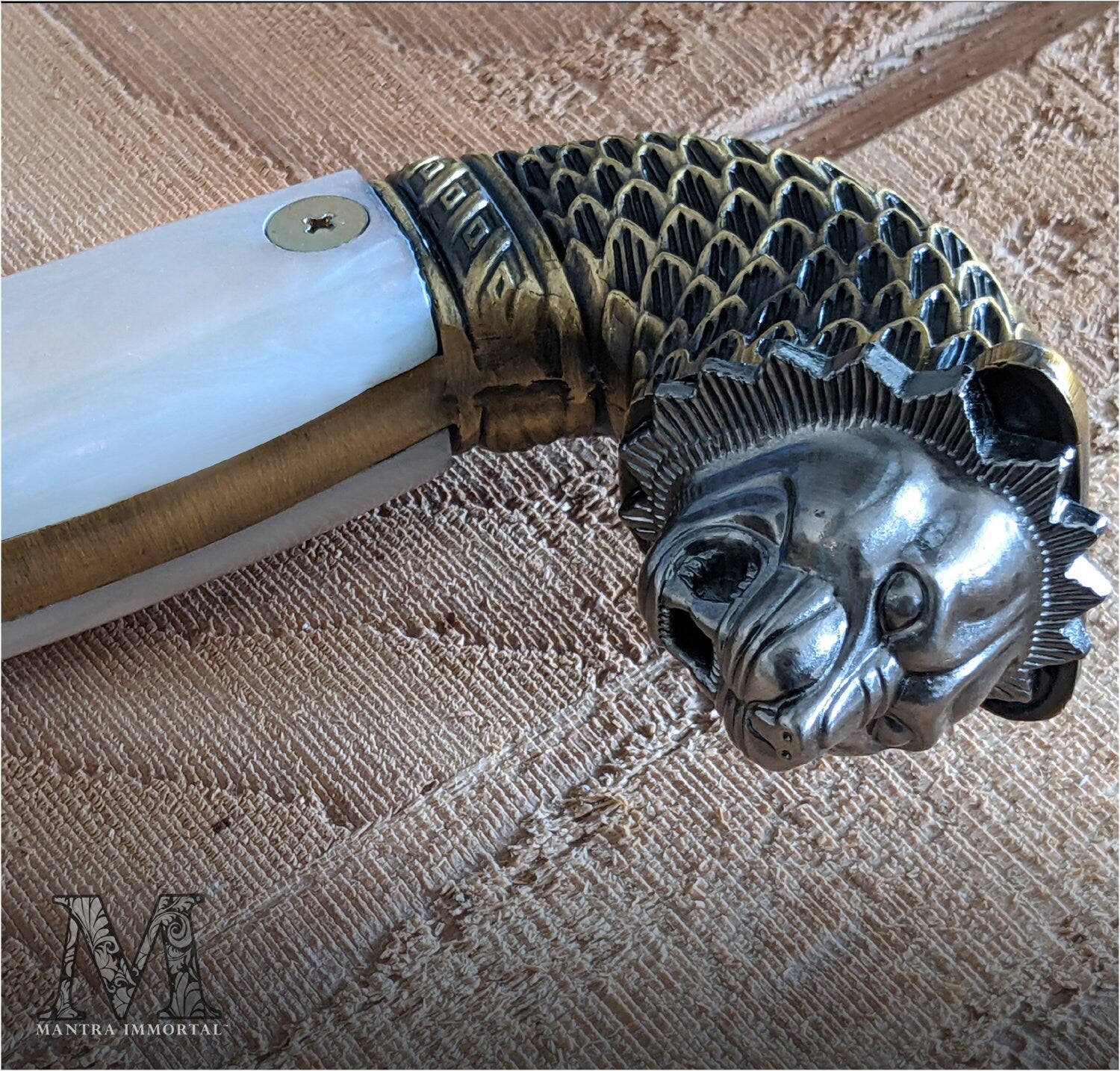The image is a professionally taken, full-color photograph, most likely captured under indoor artificial lighting. The background features a white cloth draped over what appears to be a brown wooden table. In the lower left-hand corner, there is a prominent letter "M" and the words "Mantra Immortal."

The focal point of the image is a detailed hilt, which is part of a sword or potentially the top of a cane. The handle is white with a visible screw securing it. Adorned in gold trim, the handle curves slightly upward. The most striking element is the silver head of a snarling cat, possibly a lion. This head features an open mouth, exposing sharp teeth and a ferocious expression, complete with a triangular-shaped mane. Below the cat's head is a gold portion resembling scales, adding to the ornate appearance.